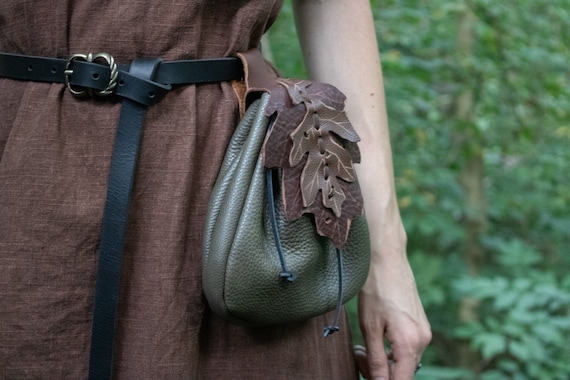The image showcases a close-up of a woman's waist, highlighting a distinct green leather pouch. She is adorned in a brown linen dress cinched with a black leather belt featuring a muted, steel-colored buckle. This intricate pouch, attached to the belt, is the main focus of the photograph. It is tear-shaped and olive green, with black leather ties dangling down. Its flap closure artfully resembles two layered brown leaves. The woman's left arm, bare and relaxed, extends behind the pouch. The background, slightly blurred, reveals a dense forest scene with tree trunks, lush green bushes, and an abundance of leaves, enhancing the rustic and natural atmosphere of the image.